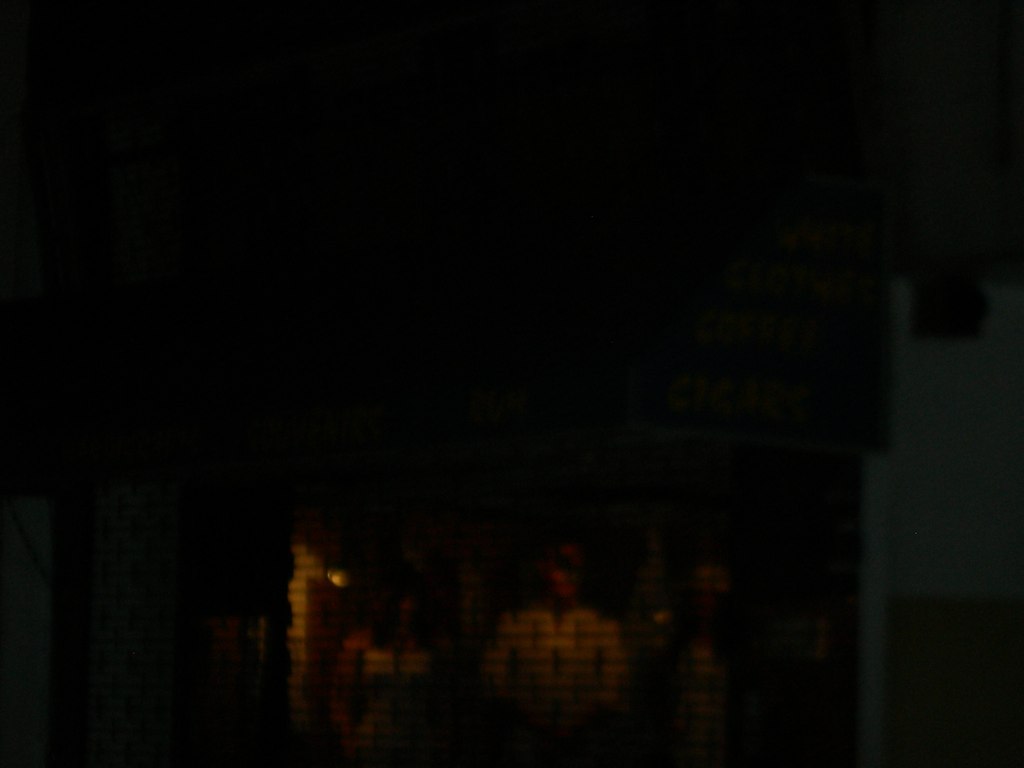In this dimly lit and blurred photograph, a multi-story building is barely discernible in the darkness. On the ground floor, behind an iron grate or gate, stands a man facing forward. His white shirt contrasts with the surrounding shadows, with a faint light illuminating him from a source mounted on a brick wall to his left. His facial features remain obscured by the darkness, but a sliver of light catches him. The man appears to have his hands in his pockets.

Next to him stands a woman with long, dark hair, wearing a strapless white dress that reveals her bare arms resting at her sides. Her presence brings a striking contrast to the gloom, her dress faintly catching the available light. To the right of the man, shrouded deeper in the shadows, another person seems to lurk, their form barely distinguishable from the darkness around them.